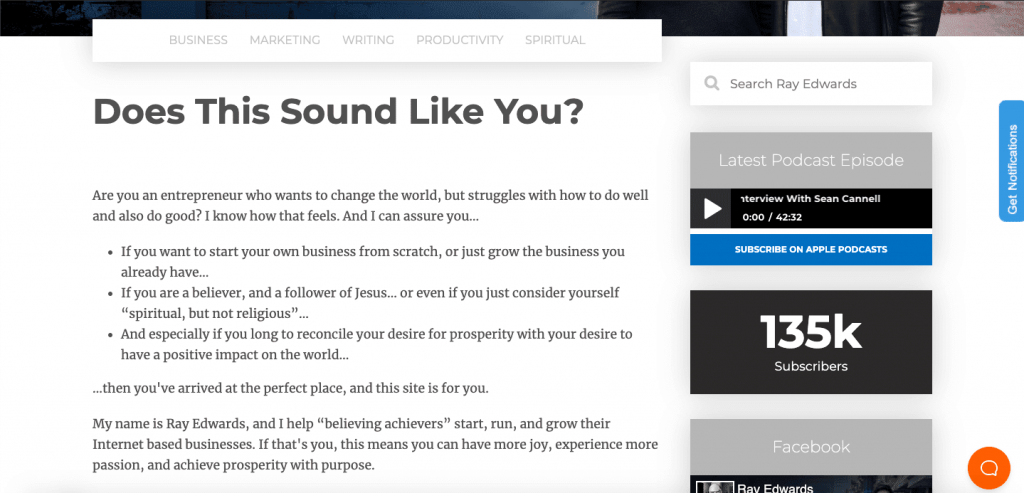This screenshot features a header with a color scheme of gray, black, and tan. Below the header, there is a white text box containing various topics listed in black text: business, marketing, writing, productivity, and spiritual. Beneath this list, a message addressed to readers begins with the question, "Does this sound like you?" The message continues, inviting entrepreneurs who aspire to make a meaningful impact on the world yet struggle with balancing success and doing good. It offers reassurance and guidance for individuals who want to start or grow their businesses, particularly those who identify as believers or followers of Jesus, as well as those who consider themselves spiritual but not religious. The text emphasizes the possibility of reconciling the desire for prosperity with having a positive impact on the world.